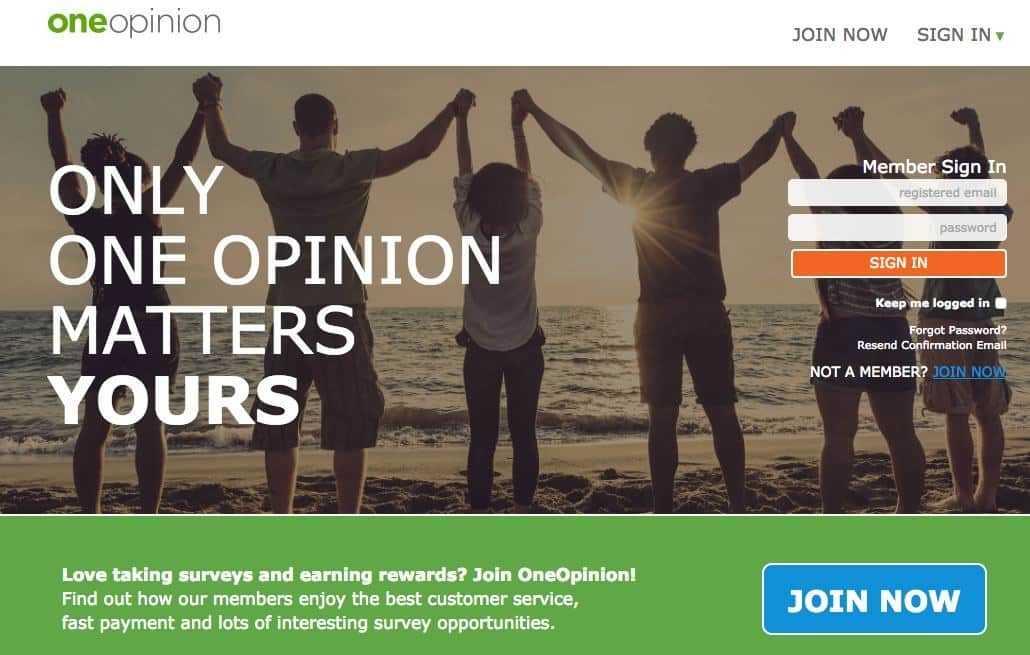In the top left corner of the image, there's a green banner with the text "One Opinion - Join Now and Sign In." Below this, a photo shows a serene scene with a bright sun shining in the background over a body of water. In the foreground, a group of people are standing hand in hand, cheering exuberantly as they face the water. 

Adjacent to the image, there's a user interface. It includes fields for registering and signing in: "Register Email," "Input Password," and an orange button labeled "Sign In." There are also options such as "Keep me logged in," "Forgot Password," and a link for "Confirmation Email."

Further down, the image urges non-members to join with a green rectangle stating, "Love taking surveys and earning rewards? Join One Opinion." It highlights benefits like "the best customer service, fast payment, and lots of interesting surveys." Additional elements include a blue rectangle with the prompt "Join Now" and a dropdown menu for signing in.

Overall, the scene blends a picturesque, uplifting moment with functional prompts for an online survey platform focused on user engagement and rewards.